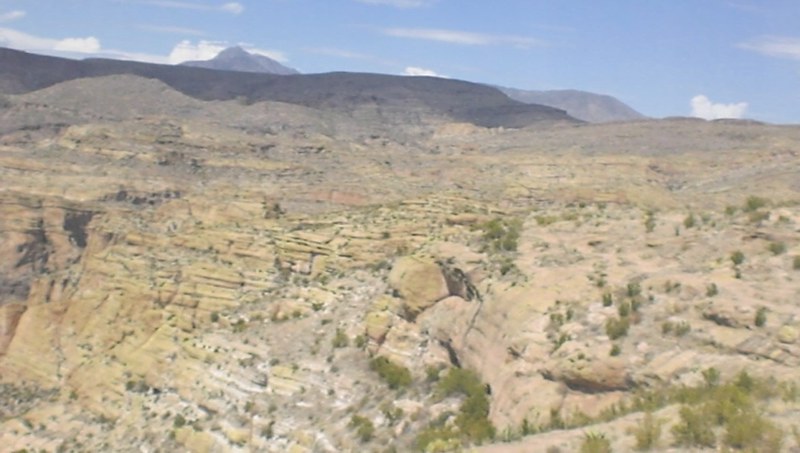The image depicts a sprawling desert landscape under a clear blue sky adorned with a few wispy white clouds. In the foreground, light tan and orangish rocks dominate, interspersed with patches of green vegetation, including bushes and sparse trees, particularly in the lower-right corner. The midsection of the image is a vast, flat plain of sandy, light brown terrain interrupted by occasional green growth. Moving further back, the landscape transitions to darker rocky hills and mountainous areas. On the left-hand side, there are dark gray hills that ascend gradually, while the right side of the image features a curved but less steep rise. The horizon is marked by a rugged, dark mountain peak that stands out against the sky. The overall impression is one of a dry, rocky expanse with minimal vegetation, captured from a vantage point that suggests the viewer is either atop a cliff or a high hill, enhancing the sense of vastness and depth.